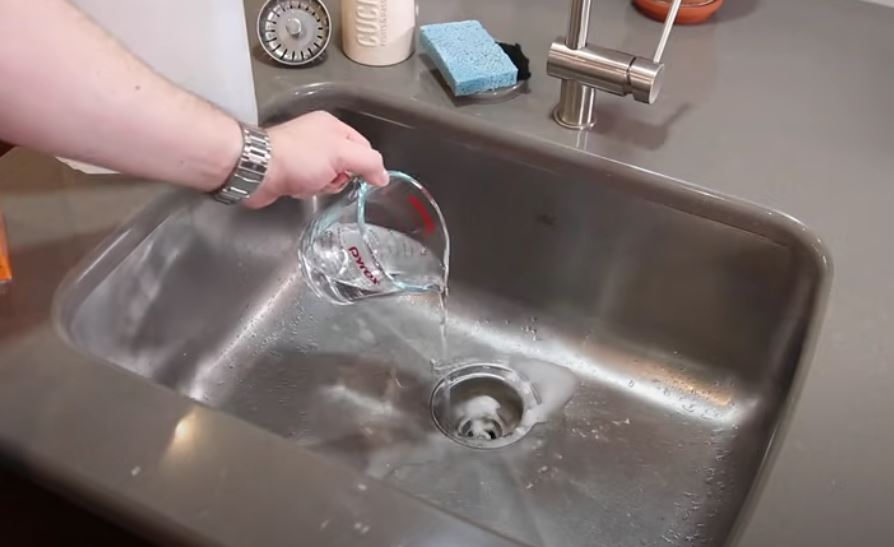In this image, a white Caucasian person with a metal wristwatch on their left wrist is pouring a white liquid from a glass measuring jug with red markings into a grey sink. The countertop around the sink is a dark grey, while the tap is silver. On the left side of the sink, there is a blue sponge and a circular drain stopper. Between the sponge and the drain stopper, there is a piece of light brown tubing labeled "C.U.C." Additionally, a clear plastic object, possibly a cutting board, is positioned to the left. Just behind the tap, there is a flat, round, orange object that appears to be an orange plate.